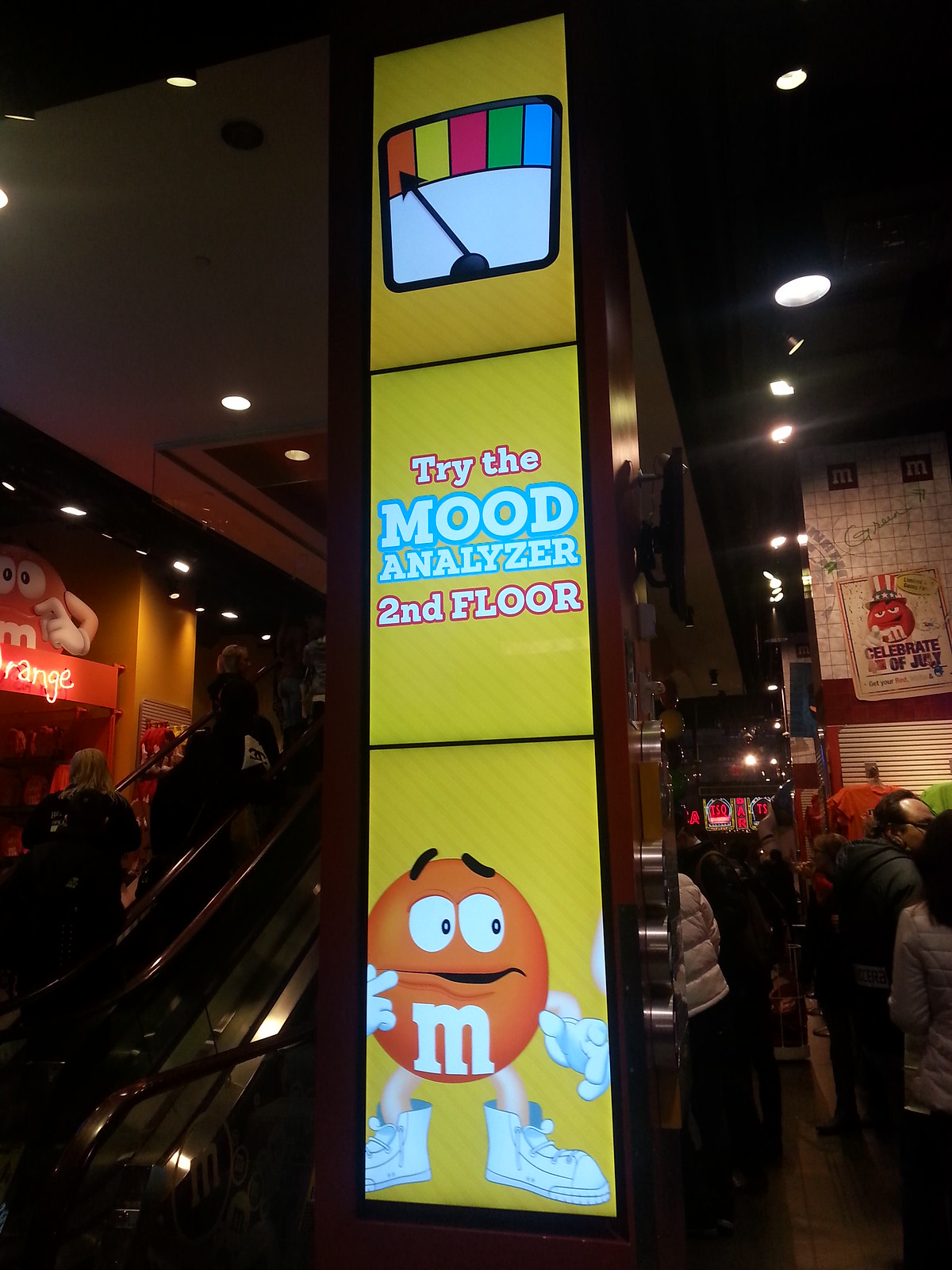The photograph captures the bustling interior of the M&M's store in Times Square, characterized by its vivid colors and lively atmosphere. Dominating the right side of the image is a large digital billboard with three sections. The top screen features a colorful meter with an arrow currently pointing to the orange section. The middle screen invites visitors to "try the mood analyzer, second floor," while the bottom screen depicts the orange M&M character looking anxious. The high-ceilinged store is filled with lights and shoppers, with merchandise such as t-shirts on the walls to the right and backpacks to the left of the escalator. Additionally, a smaller poster promoting a red M&M celebrating the 4th of July with an American Yankee hat is visible in the background. The scene is lively with people shopping and riding the escalator, embodying the energetic spirit of this famous candy store.